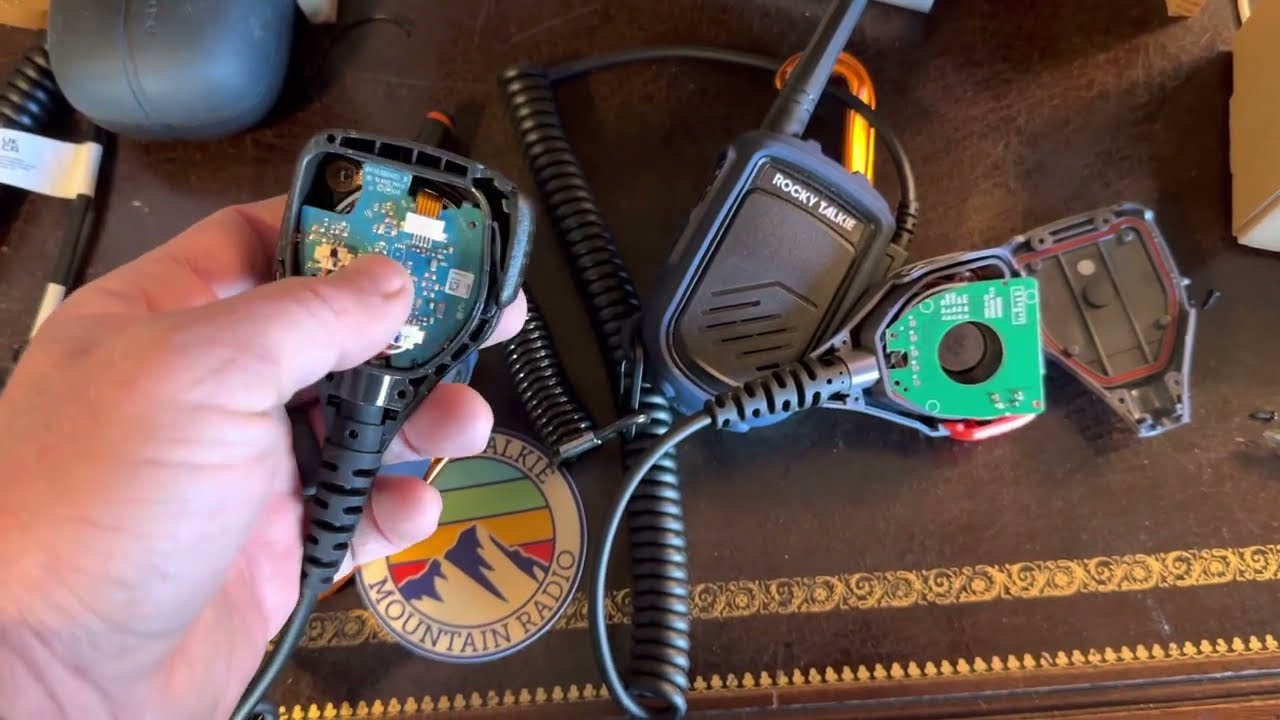The image showcases a collection of disassembled walkie-talkie parts on a decorated brown surface. Prominently placed in the center is a black plastic-framed walkie-talkie labeled "Rocky Talkie," featuring an antenna angled upwards to the right. This device has a distinctive black rectangular speaker with curved bottom edges and etched downward-sloping lines. Flanking the central piece are two similar walkie-talkies that have been opened to reveal their inner circuitry. The right-side device exposes a green circuit board adorned with illegibly small white lettering and is accompanied by its black plastic back cover with an amber trim resting beside it. The left side displays a close-up of a Caucasian hand, with short fingernails, holding another dismantled walkie-talkie, revealing a blue circuit board with visible copper lines. Beneath the hand lies a circular badge that reads "Mountain Radio," encircling an etching of a mountain peak, accompanied by colorful horizontal stripes—red, yellow, green, and blue. The entire arrangement rests on a brown surface with intricate designs, featuring slightly tilted horizontal lines and patterns resembling swirls and clovers. The scene seems to be set indoors, possibly in an electronics room.